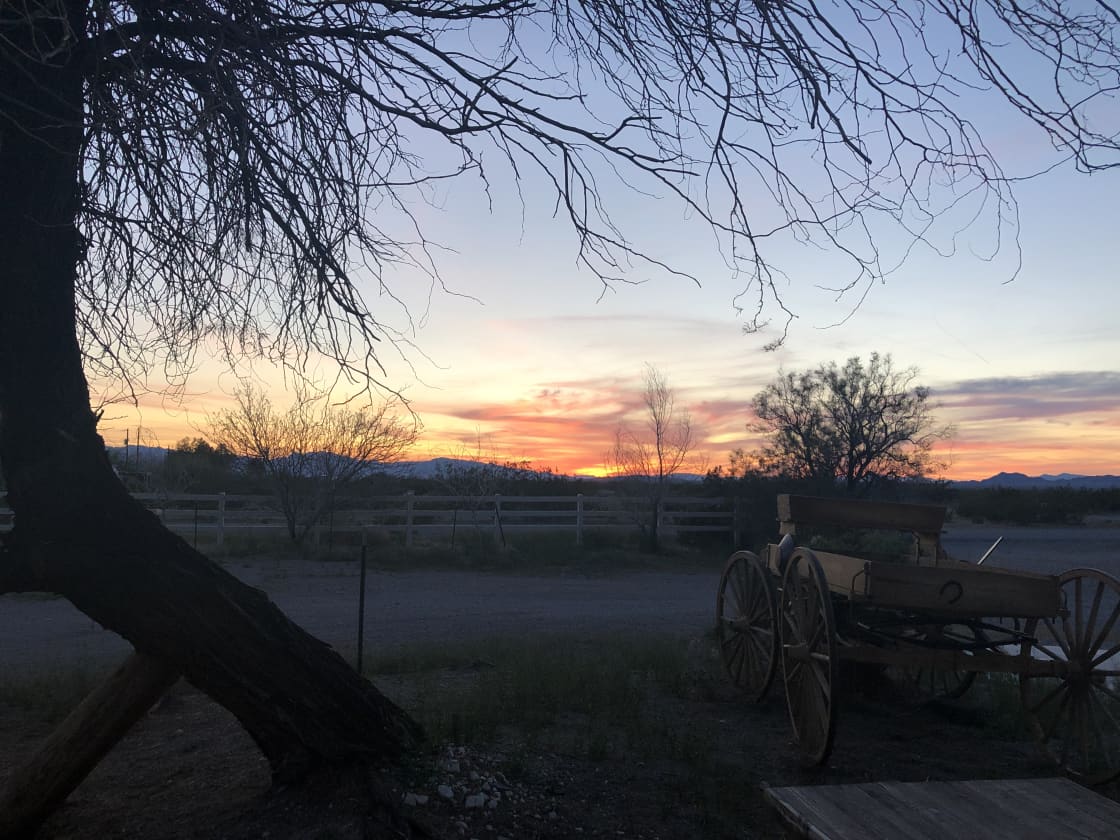The photo depicts a serene rural landscape at sunset, casting a warm golden hue across the scene. The sky transitions from blue hazy white at the top to rich oranges and purples near the horizon, adding to the tranquil ambiance. In the foreground, there is a patch of grass leading towards a large, leafless tree on the left with black, spiky branches silhouetted against the sky. 

A white, three-rail wooden fence runs horizontally across the middle of the photo, partially obscuring a paved country road. This rustic element, alongside a weathered, old-fashioned wooden buggy with spoke wheels on the right, amplifies the pastoral charm. The buggy, likely horse-drawn, sits with just its frame and four wheels, exuding an antique flair.

Other dark, shadowy trees are visible in the distance, creating silhouettes in the fading light. The overall color scheme is dominated by earthy browns and greens, complemented by the striking purple and reddish hues of the setting sun, partly veiled by a cloud. The simplicity and tranquility of this country scene are captivating, capturing a moment of quiet beauty at day's end.